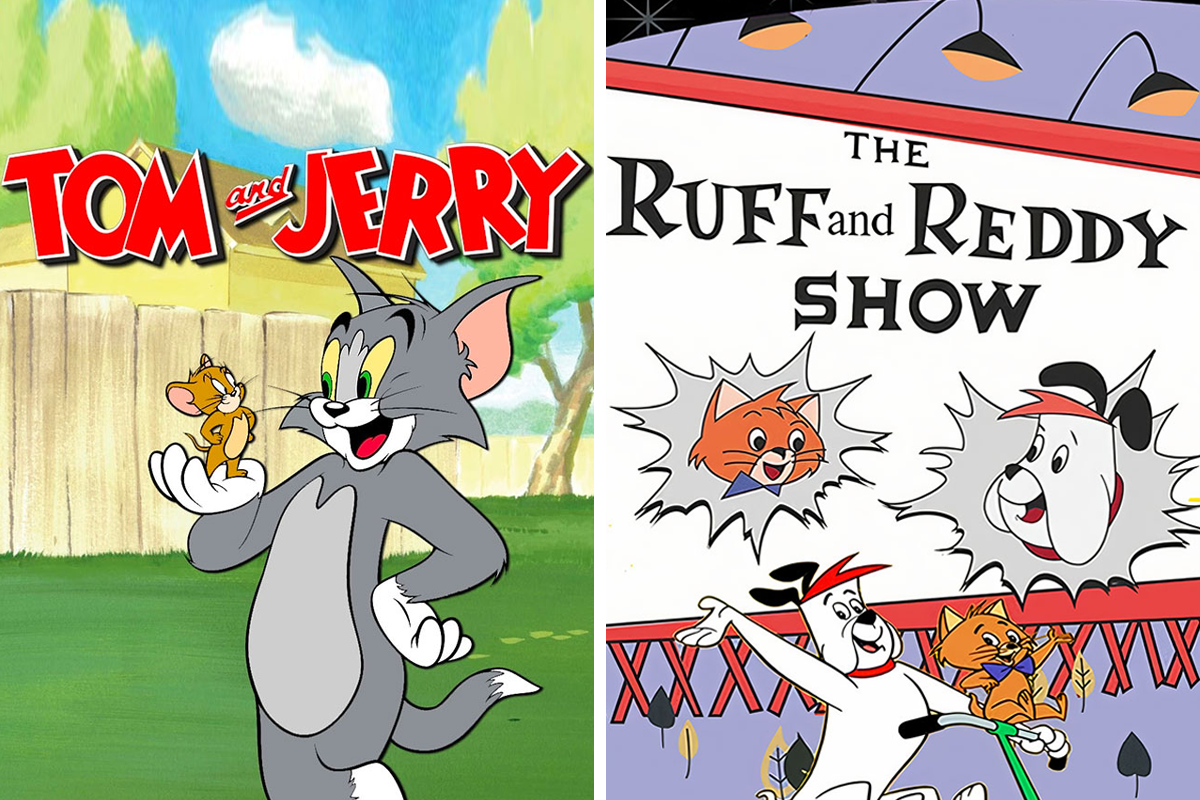The image displays two side-by-side illustrations of classic cartoon characters. On the left side, it features the well-known duo from "Tom and Jerry." Tom, the large gray cat, stands on a green lawn with one arm on his hip and his legs crossed. His other arm, extended with his palm open, holds Jerry, the small brown mouse. Both characters are looking at each other with Jerry standing confidently with both hands on his hips. The background showcases a fence, some trees, and a blue sky with a single cloud. The image is labeled "Tom and Jerry."

On the right side, the image depicts "The Ruff and Reddy Show." It shows a white bulldog with black ears and orange-red hair alongside his friend, a small brown cat wearing a blue bow tie. Both characters are looking at each other, and they appear on a white billboard with a red trim. Below, they are also shown in action: the bulldog is riding a green bike with one hand on the handlebars and the other hand raised, while the cat sits on the handlebars with one hand on its hip and the other hand up. Both characters are smiling. The background includes elements like a gray explosion pattern and small beige flowers, enhancing the vintage feel of the scene.